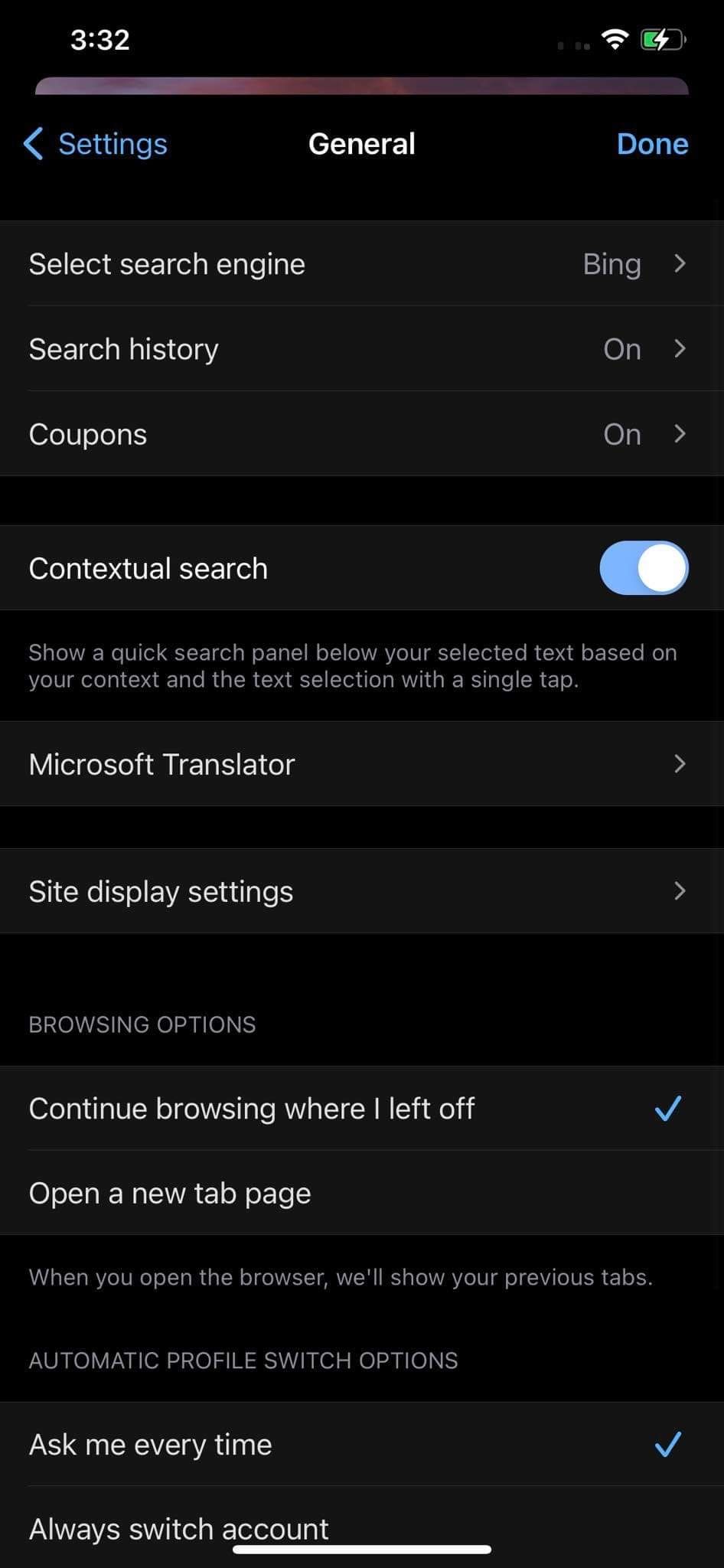The image is a vertical, rectangular screenshot with a black background, possibly taken from a cell phone. At the top, the status bar displays the time as 3:32 in white text on the left side. On the right side of the status bar are icons indicating full Wi-Fi signal strength and a charging battery. 

Below the status bar, a purple horizontal bar separates it from the rest of the image. The screen title 'Settings' is displayed at the top, with a 'General' tab selected. To the left of 'Settings,' there's a left-pointing arrow. 

The first section shows options under 'General':
- 'Select search engine' with 'Bing' currently selected, indicated by an arrow to the right.
- 'Search history,' which is turned on, again indicated by an arrow to the right.
- 'Coupons,' also turned on, with an arrow to the right.

In the next section, the 'Contextual search' option is turned on. This feature provides a quick search panel based on your context and text selection with a single tap. 

Following that, there are additional options with arrows pointing to the right:
- 'Microsoft Translator'
- 'Site display settings'

In the 'Browsing options' section:
- 'Resume browsing where I left off' is checked.
- 'Open a new tab page' is listed below.